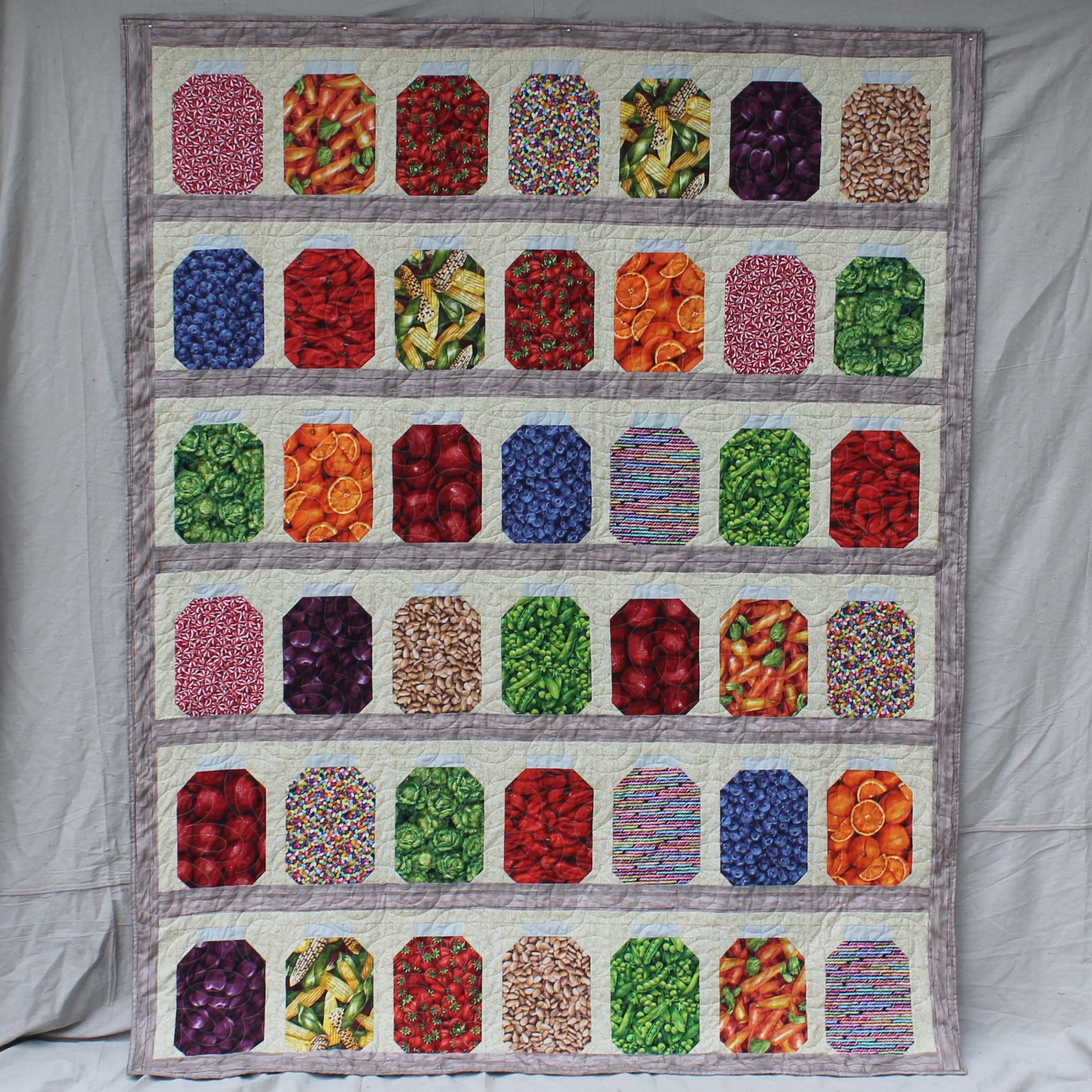This image features a colorful quilt displayed against an off-white tarp background. The quilt is divided into six horizontal rows, each containing seven elongated octagonal sections, giving the appearance of jars neatly arranged on a shelf. Each "jar" is filled with a detailed illustration of various fruits, vegetables, and nuts. The images include carrots, strawberries, oranges, corn, blueberries, tangerines, peppers, coffee beans, and some unidentified red items, among others. The illustrations repeat irregularly throughout the quilt, creating a vibrant and visually appealing pattern. The quilt’s border is a light brown color, adding a subtle frame to the diverse array of produce depicted in each section.